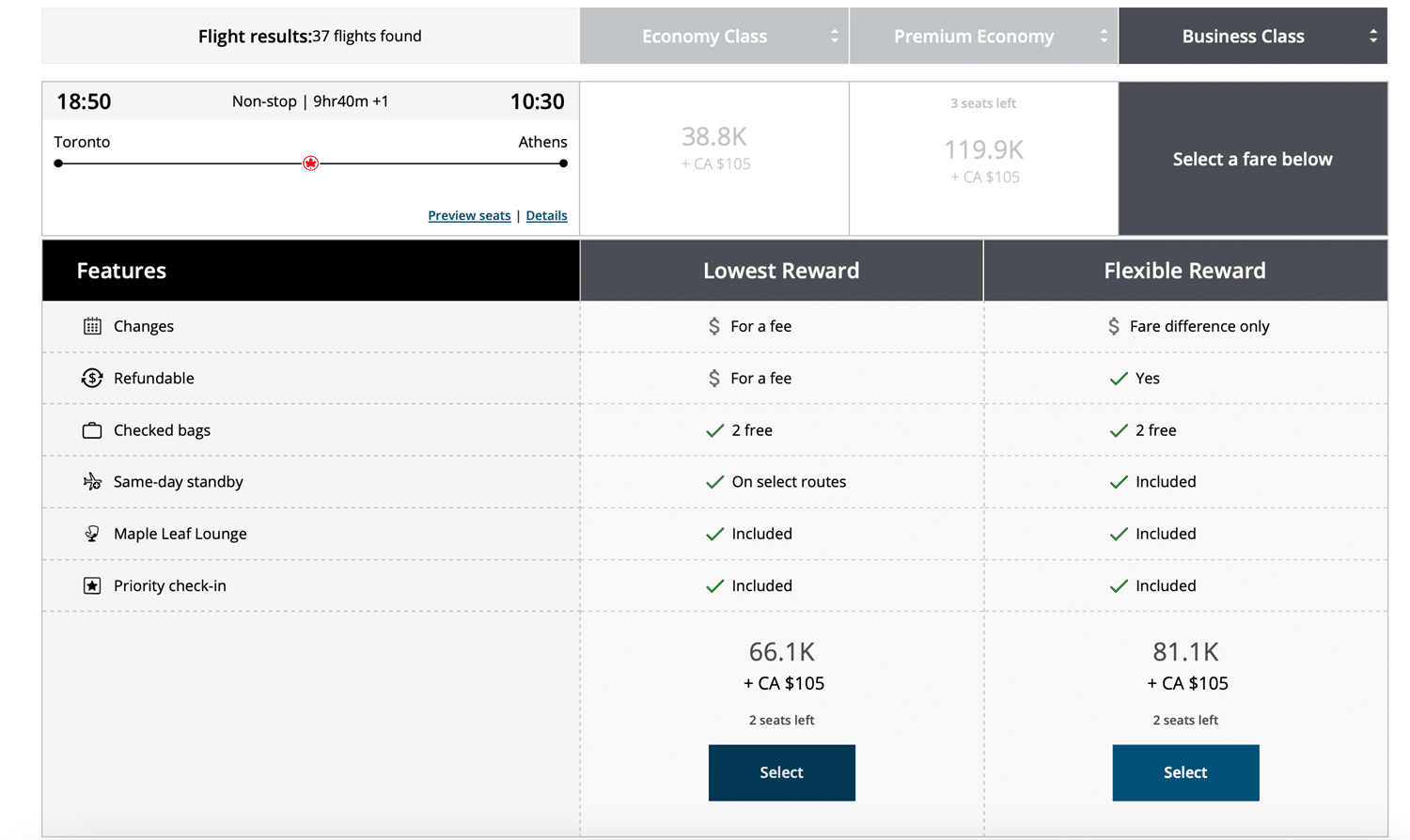The image shows a flight booking interface against a white background. The top section features a light gray box with the heading "Flight Results," indicating that 37 flights were found. The search criteria include non-stop flights at 18:50 and 10:30, specifically from Toronto to Athens. 

Below this, a black line with a red circle is featured prominently, followed by a black box titled "Features." Several amenities and options are listed underneath this heading.

To the right, the interface is divided into various fare classes, starting with light gray sections for Economy Class and Premium Economy, transitioning to a darker gray section for Business Class. Above these sections, a note reads "Select a fare below."

Within each fare class, options are detailed with accompanying benefits marked by checkmarks. In the Economy Class, for example, the "Lowest Reward" option is priced at 66.1k points plus CA $105, with only two seats remaining. A blue "Select" button is available for this choice.

The "Flexible Reward" option requires a fare difference only, totaling 81.1k points plus CA $105, also with two seats left. This section also features a prominent blue "Select" button.

This meticulous layout provides a comprehensive overview of available flights, fare classes, and associated options for travelers seeking routes from Toronto to Athens.